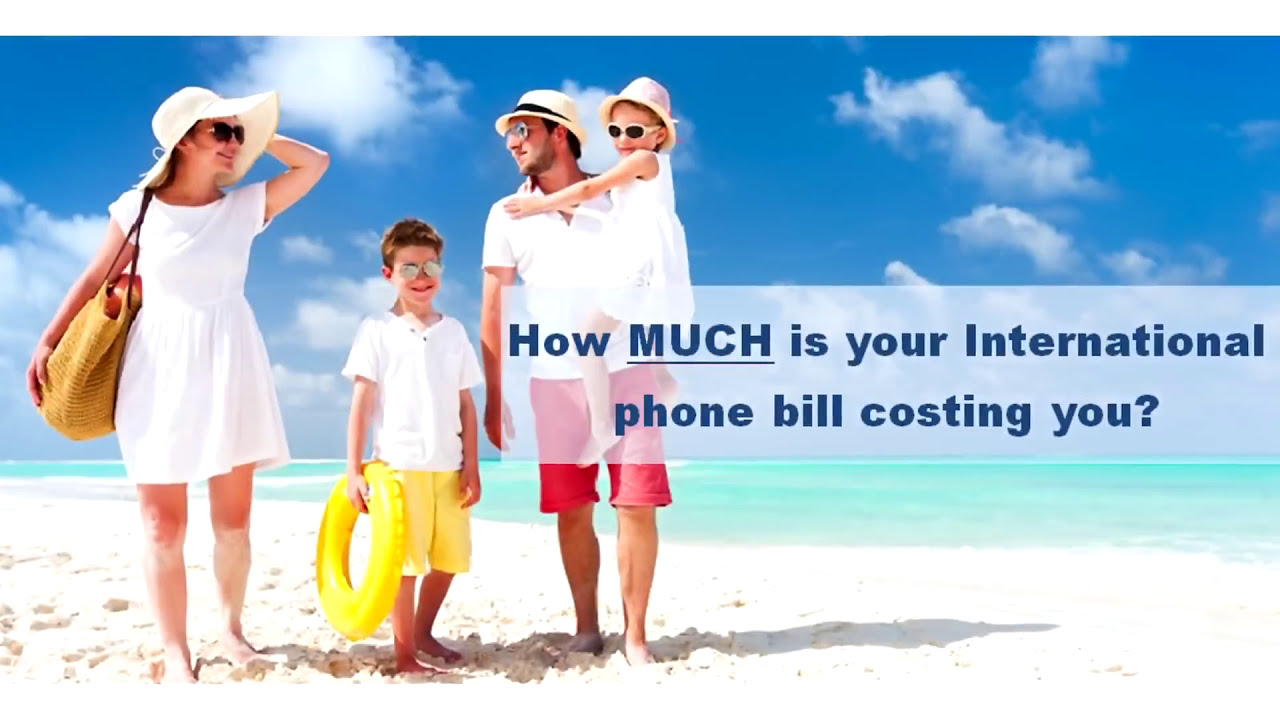This vibrant advertisement for international phone service captures a serene beach scene with a family of four standing on a brilliantly white sandy shore beneath a radiant blue sky with feathery white clouds. The family, consisting of a man, woman, young boy, and girl, is positioned on the left side of the horizontal rectangular image. All members are dressed in white attire, with the boy also donning yellow shorts and the man in red shorts. The woman, in a white bonnet-style hat and short sleeve dress, stands on the left, next to the boy who holds a circular yellow raft. The man, wearing a straw bucket hat with a black ribbon, is holding the girl who matches her mother's white sundress and straw hat. All are wearing sunglasses and smiling, exuding a sense of joy and relaxation.

Across the middle-right section of the image, blue text reads, "How much is your international phone bill costing you?" spread over two centered lines inside a semi-transparent gray rectangle. The overall scene is bathed in a supernatural vibrancy, giving the beach and sky an idyllic and inviting quality, perfectly catering to the advertisement's intent.